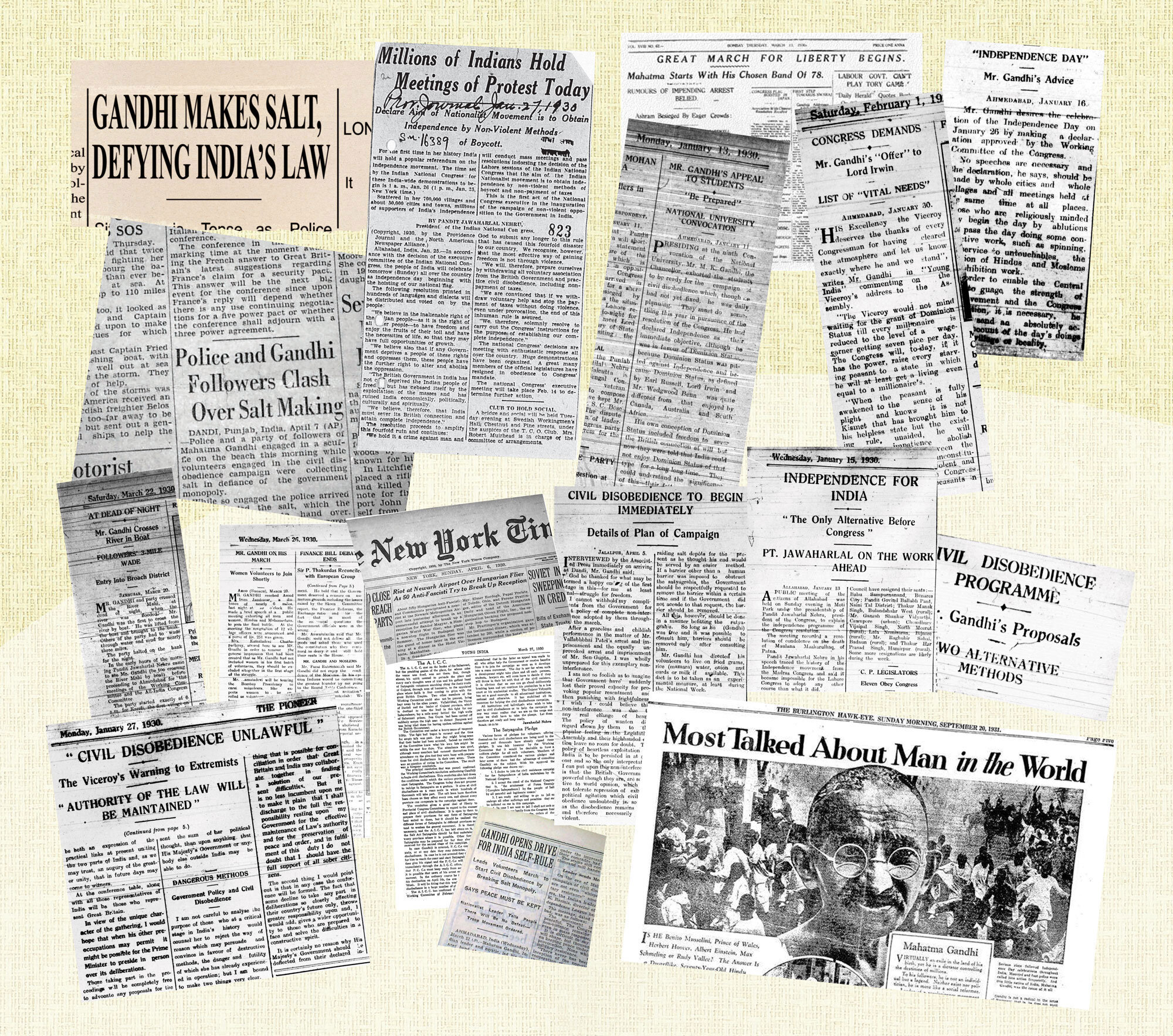The image showcases an assortment of approximately 12 to 20 old newspaper clippings laid upon a two-tone background, transitioning from yellow at the top to whitish tan at the bottom. This collection prominently features articles about Mahatma Gandhi. In the top left corner, a clipping with a brownish background boldly states, "Gandhi Makes Salt, Defying India's Law." Just to its right, headlines such as "Millions of Indians Hold Meetings of Protest Today," "Great March for Liberty Begins, Congress Demands Mr. Gandhi's Offer to Lord Erwin," and "Independence Day, Mr. Gandhi's Advice," can be observed. The bottom right corner hosts a significant article titled, "Most Talked About Man in the World," accompanied by either a photograph or illustration of Gandhi's face with the publication detail, "The Burlington Hawkeye, Sunday Morning, September 20, 1933." Additional clippings include mentions of the New York Times and titles like "Civil Disobedience Unlawful" from The Pioneer dated Monday, January 27, 1936. The clippings collectively narrate key moments and movements led by Gandhi, encapsulating his role in India’s struggle for independence.